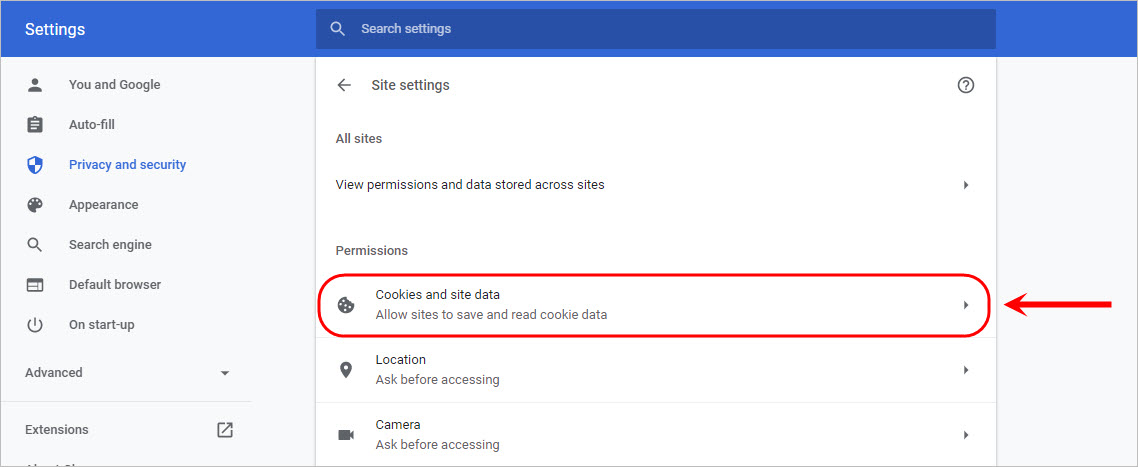This screenshot captures the 'Settings' page of the Google Chrome browser.

At the top, there's a prominent blue bar with the word "Settings" written in white. Just below this header is a darker blue section housing an input field for searching settings, marked by a magnifying glass icon on the left.

Several options are listed below this search field, each accompanied by a distinct icon: 
1. "You and Google" (person icon)
2. "Autofill" (clipboard icon)
3. "Privacy and Security" (shield badge icon) - Currently selected and highlighted in blue.
4. "Appearance" (painter's palette icon)
5. "Search Engine" (magnifying glass icon)
6. "Default Browser" (web browser icon)
7. "On Startup" (power button icon)
8. "Advanced" and "Extensions" (underneath, partially cut off)

The focus is on "Privacy and Security," featuring further options:
1. **Site Settings** - A back arrow directs to this.
2. **All Sites** - Displays a list of all sites.
3. **View permissions and data stored across sites** - Accompanied by a closed toggle/dropdown.
4. **Permissions**:
   - **Cookies and Site Data** - Icon of a cookie with a bite taken out. The description says, "Allow sites to save and read cookie data."
   - **Location** - Icon of a map pointer arrow. The description says, "Ask before accessing."
   - **Camera** - Icon of a video camera. The description says, "Ask before accessing."

Encircling "Cookies and Site Data" is a red oval (capsule), with a red arrow pointing towards it from the right side of the screen, emphasizing this section.

The narrative concludes with the phrases beneath the location and camera permissions, affirming "Ask before accessing"safety settings.